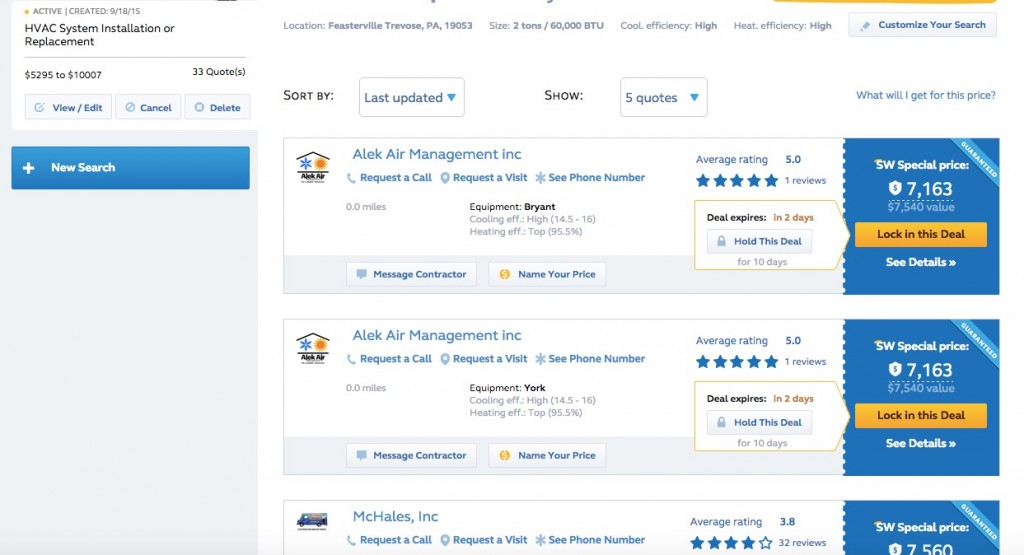The image depicts a search result for HVAC system installations or replacements, with prices varying from $5,295 to $10,007 and a total of 33 quotes available. The highlighted result is from ALEC Air Management INC, which offers various options such as requesting a call, scheduling a visit, or viewing the phone number. This contractor has an average rating of 5 stars based on a single review. An exclusive offer is listed at a special price of $7,163, with options to lock in the deal, view more details, message the contractor, or propose your own price. The location is specified as Feasterville-Trevose, PA 19053, featuring a unit size of 2 tons and 60,000 BTU. The system is noted for its high efficiency in both cooling and heating.